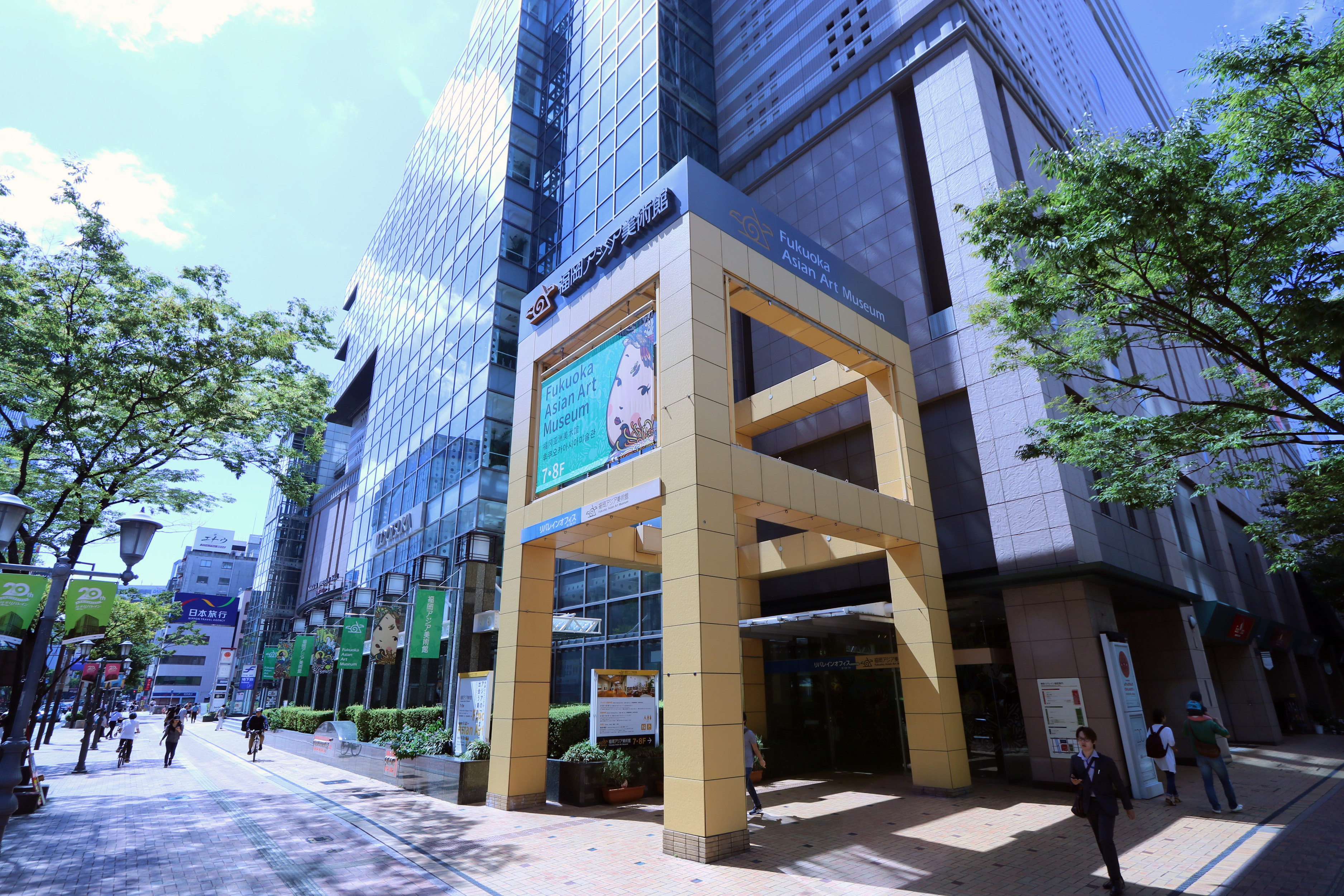The photograph captures a bustling city street, dominated by a striking tall office building composed of reflective glass square windows. The building, primarily dark gray and white, features prominent yellow pillars at its front, adorned with an animated picture of a child. The scene is bathed in sunlight under a clear, blue sky with sparse white clouds, indicating a warm, pleasant day. The street in front of the building is lively with activity; several people are visible, including a woman in a black jacket and blue collared shirt walking towards the camera, a family with members wearing white and green shirts walking away, and a cyclist navigating the street. Green banners hang from the light posts lining the walkway, complemented by vibrant trees with purple blossoms on both sides. This dynamic urban environment, possibly within an Asian city, is also marked by signs indicating the presence of an Asian Art Museum, enhancing the cultural ambiance of the scene.